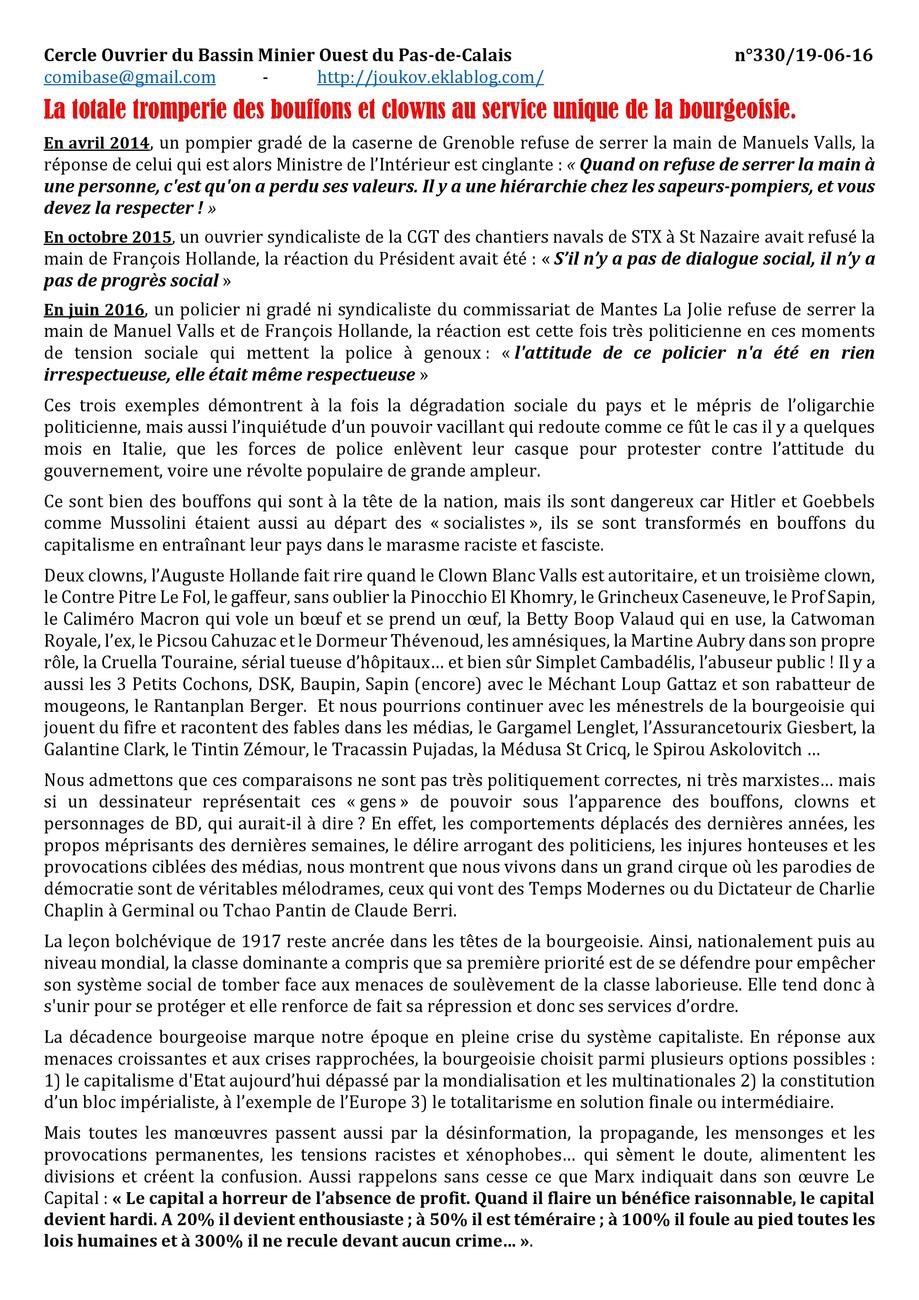The document is a text page written in French, predominantly in black script on a white background. At the very top, there is a small bolded line of text in French, followed by a blue, underlined email address, comibase@gmail.com, and a blue, underlined URL, http://joukov.eklablog.com. In the upper right-hand corner, there is a notation "n° 330 / 19-06-16," indicating the date, June 16th. Below these details is a red, bolded header. The main body of the text, which occupies approximately 80% of the page, consists of ten paragraphs in block alignment. Specific dates, such as April 2014, October 2015, and June 2016, are bolded and underlined within the text. At the end of the document, there are three additional lines in bold print.